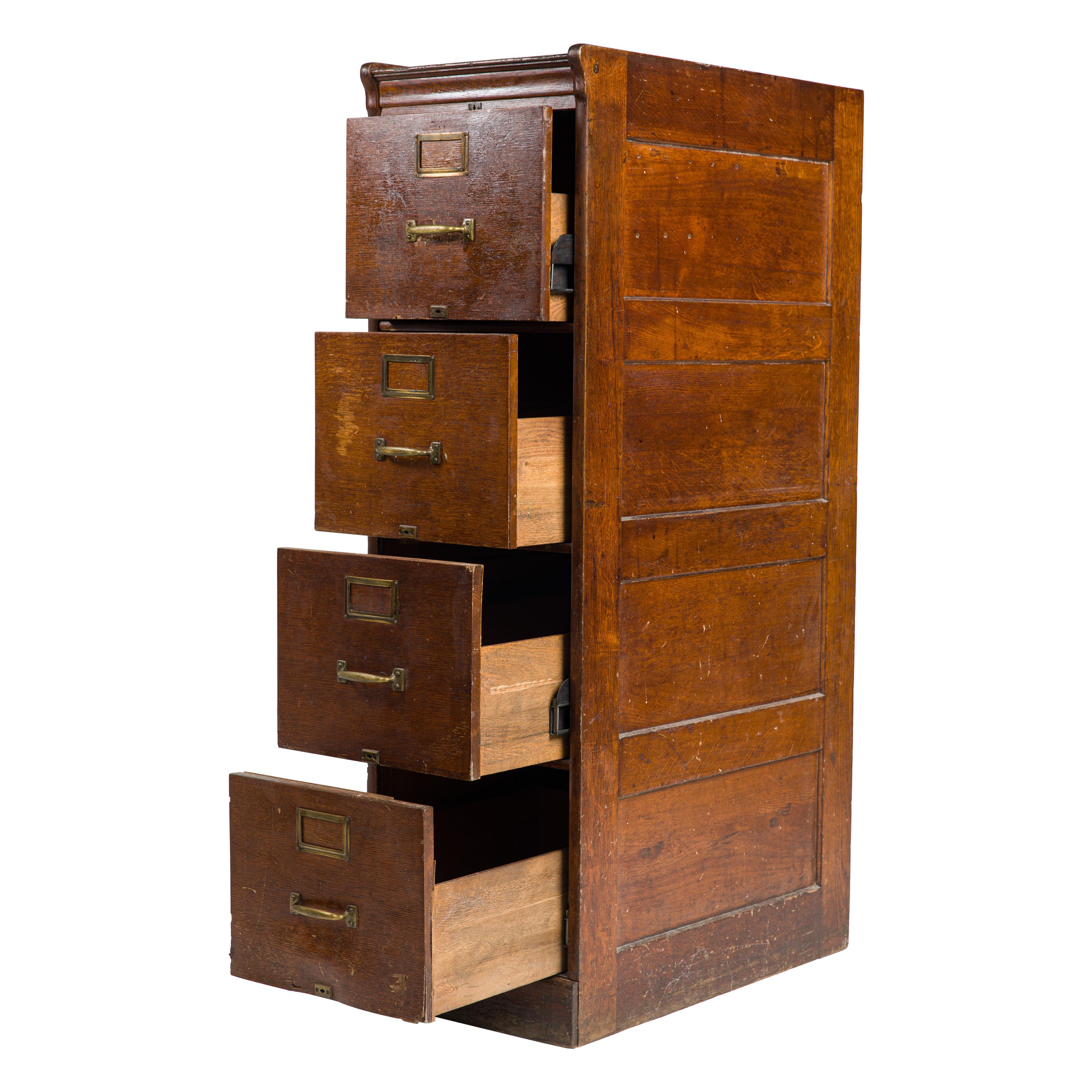This image showcases a vintage wooden filing cabinet, potentially dating back to the late 1930s to 1950s. Unlike the more common metal cabinets designed to protect documents from fire, this piece is crafted from a richly stained mahogany wood, giving it a textured and dark appearance. The cabinet features four drawers, each equipped with a brass handle and an ID card slot, currently empty. The bottom drawer is fully open, while the drawers above it are progressively less open, with the top drawer almost completely shut. Despite some scuff marks on the bottom and drawer fronts, the cabinet remains in good condition, showing typical signs of wear and tear for its age. The background of the image is entirely white, likely intended to highlight the piece for an online sale or display.